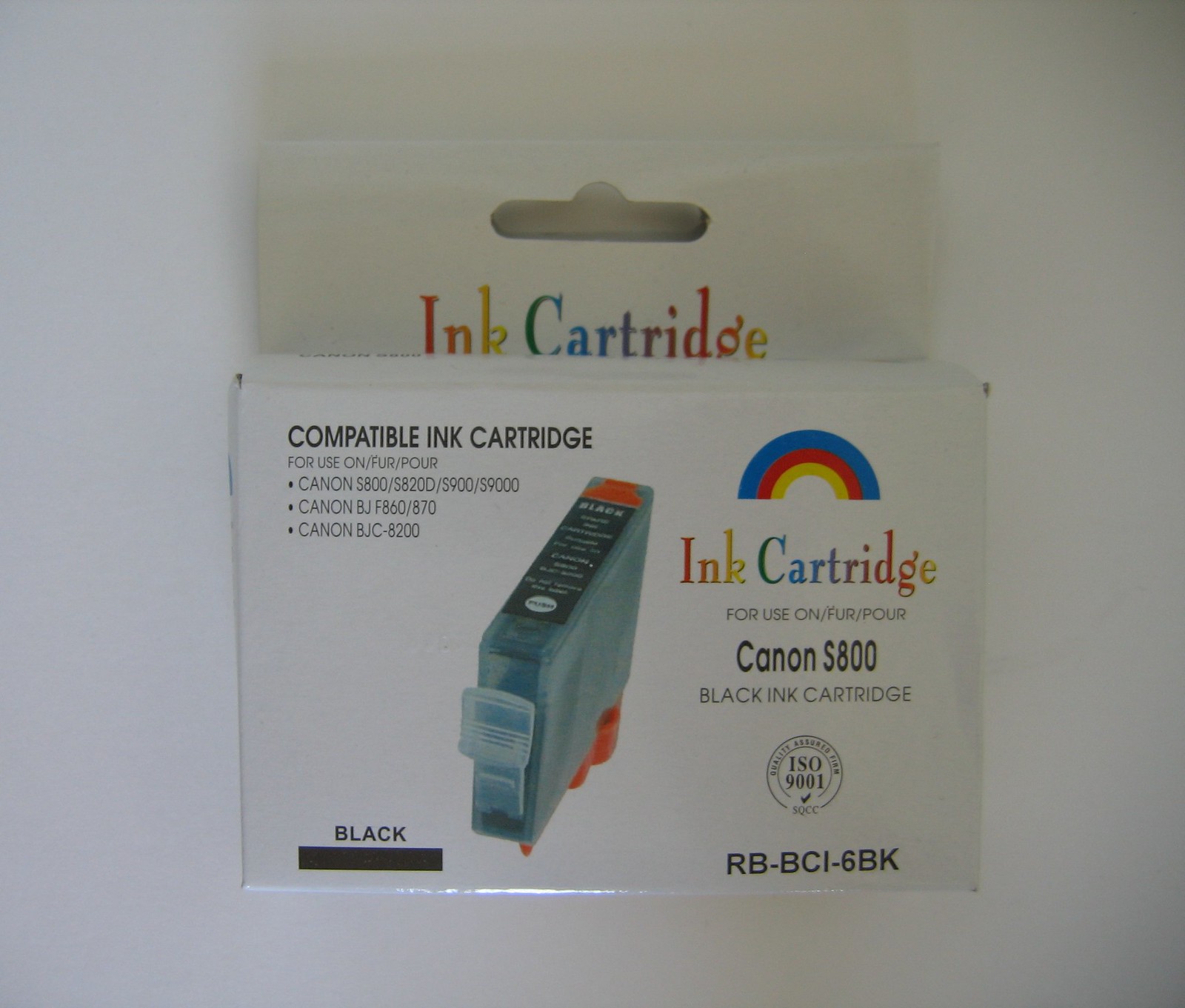The image features a sleek, white, shiny-coated cardboard package for an ink cartridge, presumably for a printer. At the top of the package, "ink cartridge" is prominently displayed in bold, multicolored font, creating a rainbow-like effect with blue, red, and yellow hues. Above this text, there is a visual rainbow emblem.

Beneath the colorful title, in clean black text, the package states that it is a "compatible ink cartridge for use on Canon S800, Canon S820, Canon S900, Canon S9000, Canon BJ F860 / 870, and Canon BJC-8200" models. It indicates that the ink color is black. Additionally, there is an image of the actual rectangular ink cartridge itself, which would be found inside the packaging.

Moreover, the package features a small circle resembling a stamp of approval, which reads "ISO 9001" signifying quality assurance. The bottom right corner of the package is marked with "RB BCI-6BK." The entire package is set against a white background, enhancing its clean and professional appearance.